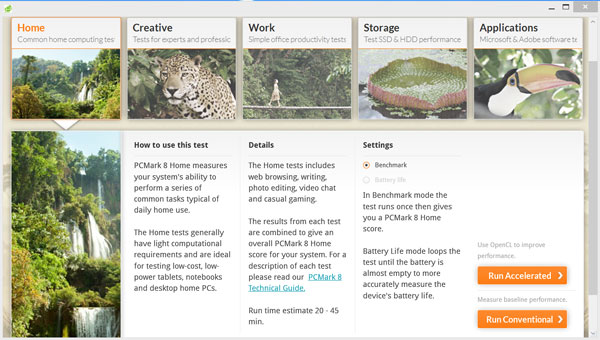This screenshot showcases a webpage with an organized layout featuring five tabs: Home, Creative, Work, Storage, and Applications, each with corresponding titles and vivid images. The Home tab, highlighted in orange, displays a picturesque rainforest. The Creative tab features a striking image of a leopard. The Work tab depicts a woman walking across a log or bridge situated over a ravine or valley. The Storage tab contains a close-up photograph of a lily pad floating on a pond. Finally, the Applications tab shows a close-up of a colorful toucan bird.

Below the tabs, a detailed chart explains the function of the PC Mark 8 Home test. It measures the system's capability to handle typical daily home tasks. The Details column lists the tasks included in the Home test: web browsing, writing, photo editing, video chat, and casual gaming. There is also a hyperlink directing to the PC Mark 8 Technical Guide, stating the test duration ranges from 20 to 45 minutes. 

Additionally, there is a Settings column set to Benchmark mode. It indicates that in this mode, the test runs once and provides a PC Mark 8 Home score upon completion. The background of the page is white, creating a clean and clear interface. On the far right side, two prominent orange buttons labeled "Run Accelerated" and "Run Conventional" invite users to initiate the test.